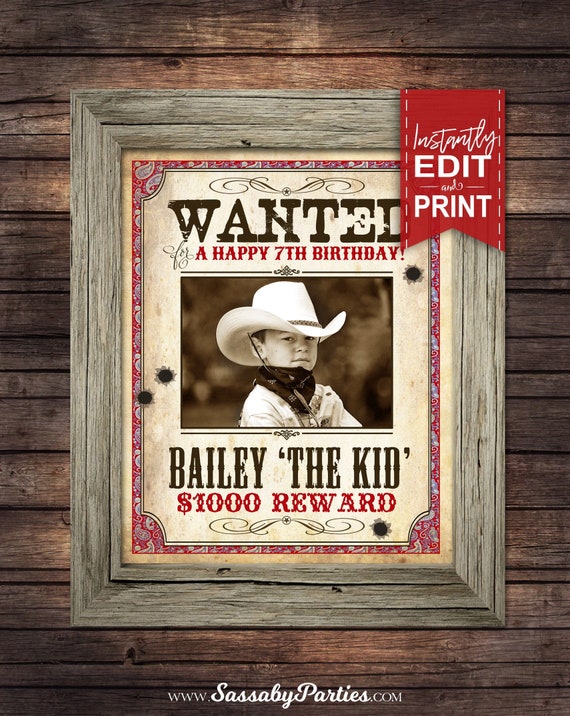This image showcases a digitally rendered, customizable birthday poster encased in a wide, gray barnwood frame. The poster features a prominent red paisley border, and at the top, in bold black text, it declares "WANTED." Just below, in smaller red text, it states "A HAPPY 7TH BIRTHDAY!" Centrally positioned is a black and white photograph of a young boy dressed in a full cowboy outfit, complete with a hat, a scarf around his neck, and a long-sleeve shirt, gazing upwards. Below his image, in large black text, reads "BAILEY 'THE KID'," followed by a red "WANTED" style "$1,000 REWARD." The poster is embellished with bullet hole graphics on either side. In the top right corner of the frame, a red vertical banner with white text reads "INSTANTLY EDIT AND PRINT," while the bottom edge of the image includes the website "www.sasabeeparties.com" in white text on a dark brown background. The image is photographed in a portrait orientation and captures the playful, western-themed birthday announcement in a realistic, product photography style.